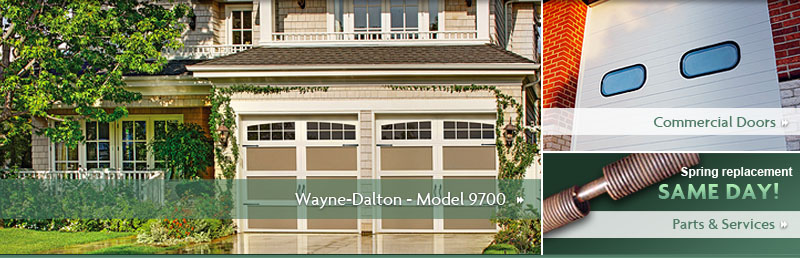**Advertisement Overview: Wayne Dalton Model 9700 and Related Services**

The advertisement features three distinct images showcasing various products and services offered. Occupying about two-thirds of the advertisement's width is the primary image of a residential house, prominently labeled "Wayne Dalton Model 9700." This section features a well-maintained tan house with brown trim, accentuated by two large garage doors at the facade. The house has multiple windows on both the first and second floors, providing a welcoming appearance. On the right side of the property, there is a white picket fence and a large tree, adding to the cozy suburban aesthetic.

To the right of this main image, two smaller photos are stacked vertically, each occupying about one-third of the advertisement's width. The first of these smaller images is titled "Commercial Doors" and displays a metallic-colored garage door installed on a commercial building. The structure itself combines red and white brick, giving it a robust and professional look.

Below the commercial door image is a green-background rectangle labeled "Spring Replacement Same Day Parts and Services." This section highlights a copper-colored spring, emphasizing the company's commitment to providing immediate parts and service solutions for garage door maintenance.